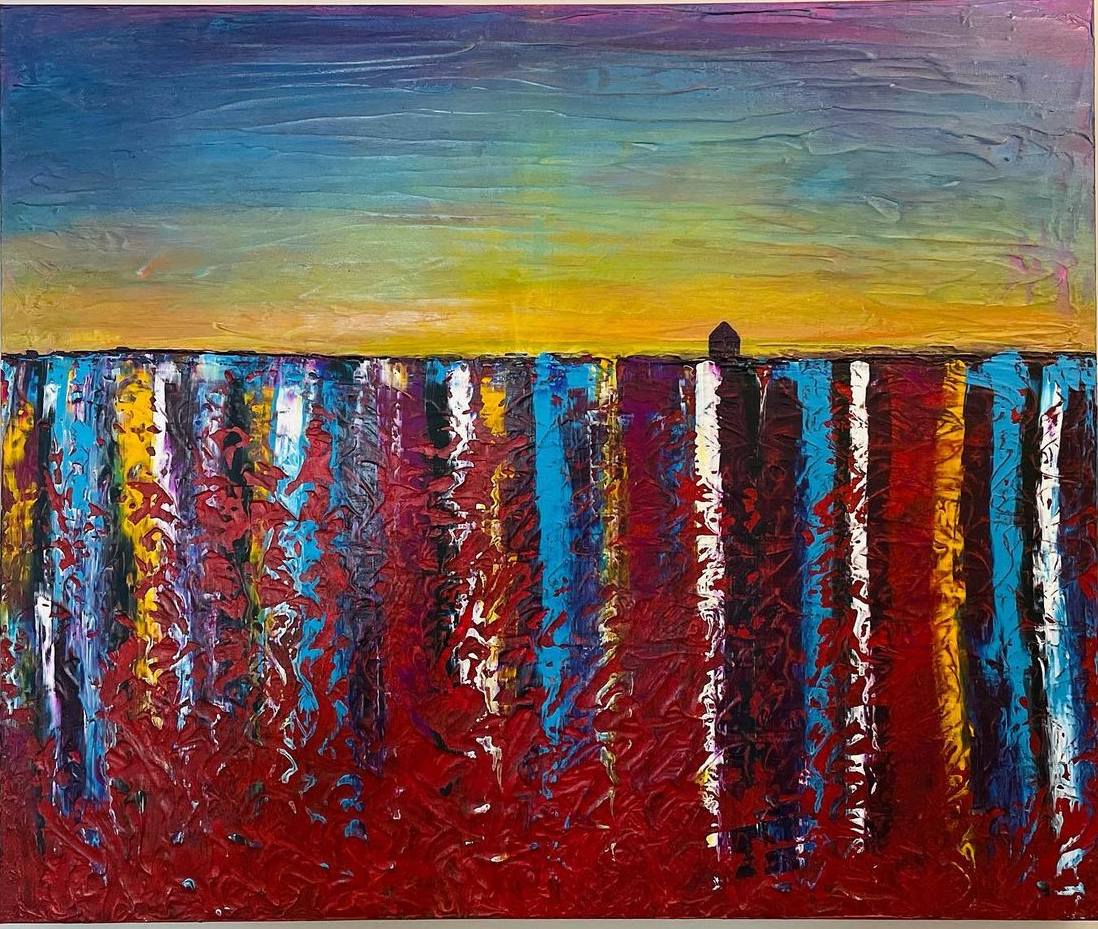This horizontal rectangular image is an abstract painting rendered on a canvas, likely an oil painting. The painting is divided into two distinct sections: the upper and lower parts, each characterized by different styles and colors.

The upper third of the painting features heavy, textured horizontal brushstrokes in a vibrant mix of colors, including primarily pink at the top, then transitioning through blue, green, yellow, orange, and touches of purple. The strokes are visibly protruding from the canvas, indicating a thick application of paint in some areas while others remain smoother.

The bottom two-thirds of the painting showcases a more structured pattern of vertical stripes, alternating in colors and spanning the width of the canvas. These stripes include shades of blue, yellow, white, and black, interspersed with red splatters that rise from the bottom of the painting. The raw, textured strokes of these vertical lines suggest a deliberate attempt to depict a weathered or rusty effect on a maroon background.

Additionally, positioned slightly past the halfway mark from the left edge of the painting, there is a small black shape that resembles a distant building. This shape has a square base and tapers off into a pointed roof, resembling a house.

With its vivid colors and contrasting textures, the painting evokes a multifaceted visual experience that draws the viewer's eye to both its structured and spontaneous elements.